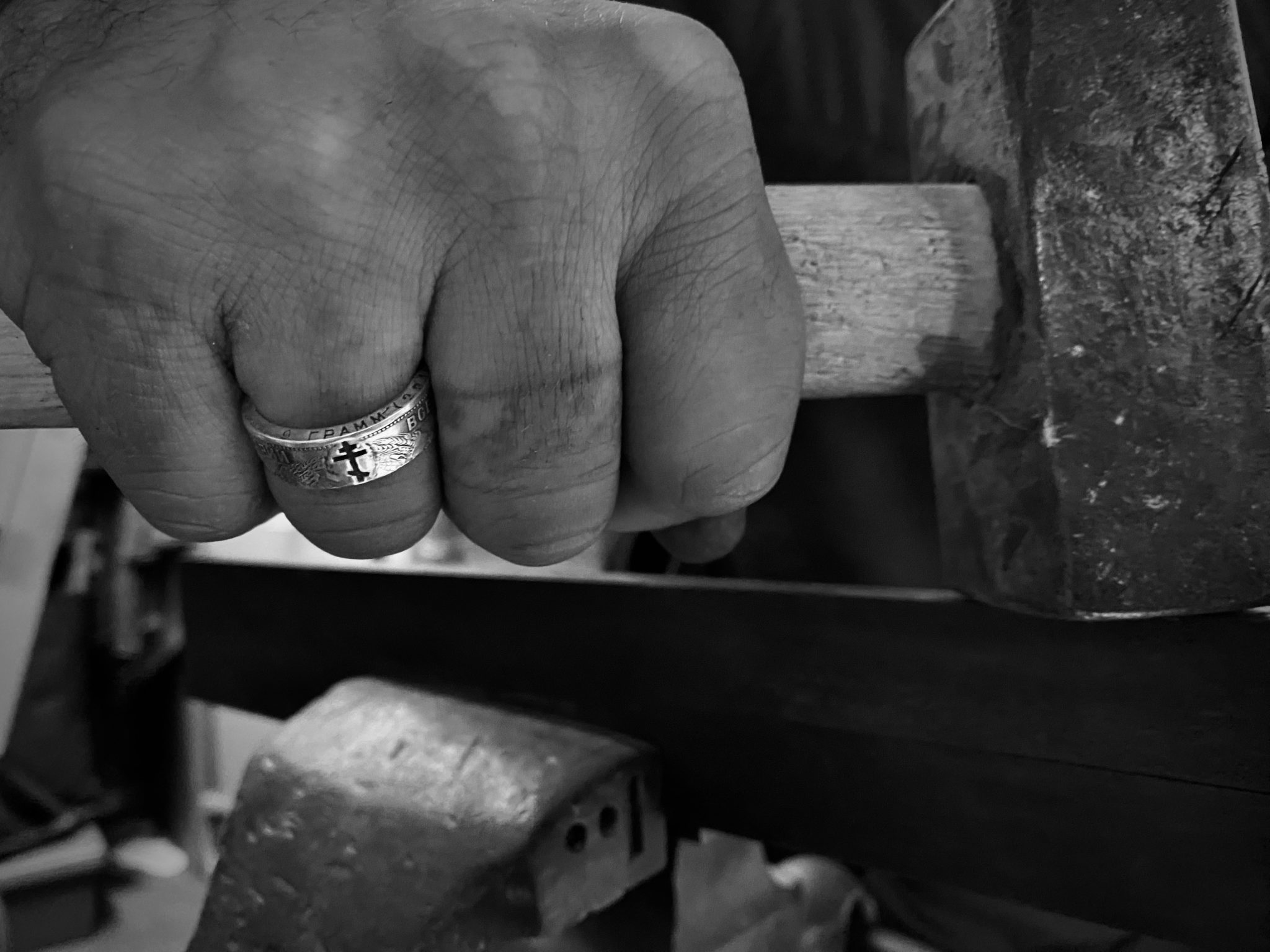This is a highly detailed black-and-white photograph capturing a close-up of a man's worn hand gripping a mallet, suggesting he might be a craftsman, possibly a metalsmith or artisan. His middle finger bears a tattoo that resembles a ring, while his ring finger sports a thick ring adorned with an Orthodox cross. The grayscale nature of the image lends a timeless quality, although it conceals the true colors of the items. The man is hammering an indeterminate piece of metal, possibly atop a wood block or in a vise. The background hints at a workshop environment, with various tools and items scattered around but remaining out of focus. The composition of the photograph is professional, with the heavy metal part of the mallet prominently positioned on the right side, directing the viewer's attention to the intense, skillful action of the craftsman.